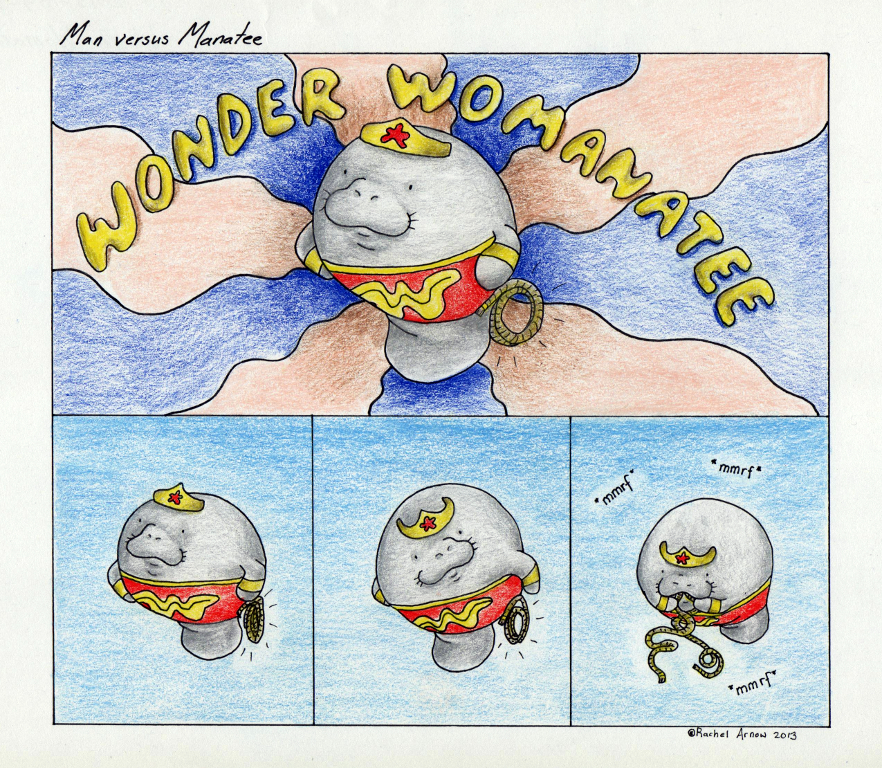This hand-drawn comic titled "Man vs. Manatee" features a humorous take on Wonder Woman with a character named Wonder Womanatee, a gray manatee in a Wonder Woman outfit. The top half of the comic showcases a large rectangular panel with a swirling blue and brown background. In bold black letters, it is captioned "Man vs. Manatee" in the upper left corner, while yellow letters spell out "Wonder Womanatee." The manatee sports a red top emblazoned with a yellow W, gold trim on the edges, a golden tiara with a red symbol, gold bangles on its fins, and a gold lasso at its hip. Radiating blue and orange accents surround this heroic sea creature.

Below this main panel, three smaller square panels depict a sequence of actions: in the first, Wonder Womanatee stands with its arms on its hips, reminiscent of a hero pose; in the second, it reaches for the lasso with its left fin; and in the third, it amusingly stuffs the lasso into its mouth. Black lettering around the edges of these panels reads "M-M-F" or "oomph," simulating the sound of eating. The background of the lower panels is filled in blue, suggesting an underwater setting.